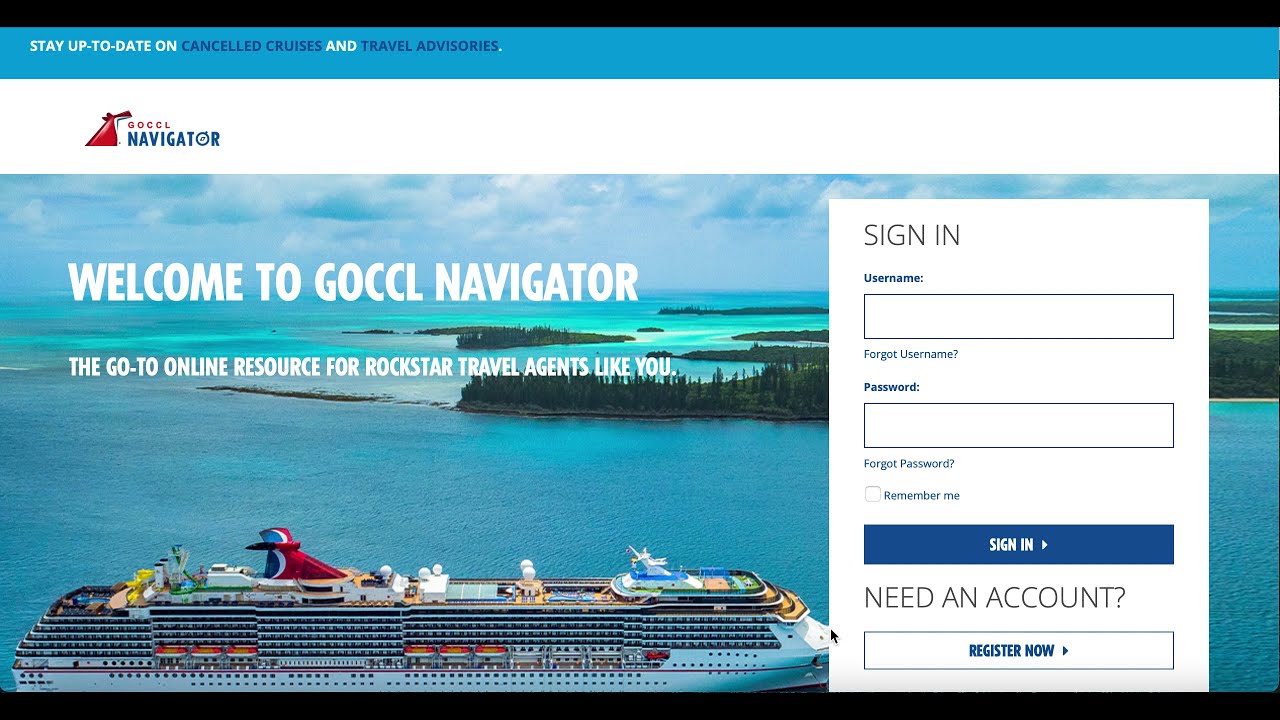A screenshot of the GeoCCL Navigator desktop app interface. The top and bottom edges are bordered by thick black bands, creating a frame for the content in between. Just below the top border, text is displayed, stating, "Stay up to date on canceled cruises and travel advisories." Beneath this message, the name of the application, "GeoCCL Navigator," is prominently featured, accompanied by a logo depicting the mainsail of a shipping vessel in red, accented with curved white and blue stripes.

The background sets a serene scene with a luxury liner cruising on a vast ocean, with lush green forestry visible on the horizon. The sky overhead is mostly clear with a scattering of clouds, enhancing the tranquil ambiance. Overlaying this picturesque setting, text reads, "Welcome to GeoCCL Navigator, the go-to online resource for rockstar travel agents like you."

To the right, a sign-in section invites users to enter their username and password, featuring a bold, rectangular sign-in button below. For new users, there is an additional white rectangular button labeled "Register Now," providing a seamless way to create an account.